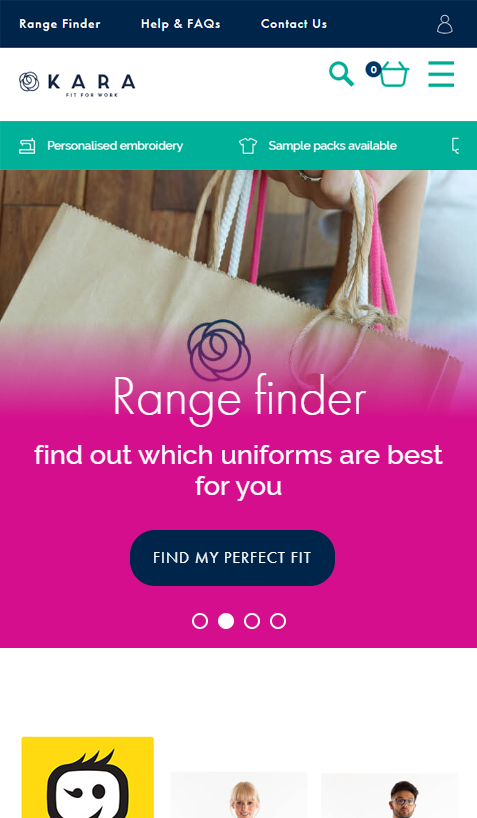This image is a phone screenshot from "Kara Fit for Work." The logo, prominently displayed, features a hand-drawn rose symbolizing the brand. At the top, a navy blue bar contains white text links to "Rangefinder," "Help & FAQs," and "Contact Us." Below is the account information, simply stating "Kara." 

A mint green banner advertises “Personalized Embroidery, Sample Packs Available.” The main section showcases a photograph of an arm holding three shopping bags. The top bag is white with bright pink accents, featuring the text "Rangefinder: Find out which uniforms are best for you. Find My Perfect Fit."

At the bottom of the screenshot, three interaction options are presented: a large yellow box with a winking emoji, followed by pictures of an actual woman and man, offering personalized assistance.